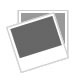The image portrays a close-up view of an object that is conical in shape, akin to either an upside-down ceramic cup, a cork from a wine bottle, or possibly an old wooden thimble. The object, appearing to be made from terracotta or dark, hand-carved wood, features a smooth surface and subtle dimples around the top. The object is positioned on its wider base with the narrower top facing upwards, resting on what seems to be a blue or denim fabric. The right side of the object bears the inscription "MALAGA" in black, all-capital letters. Additionally, there is a blue or black and gray piece attached to the left side. The overall orientation of the image is portrait, making it taller than it is wide.